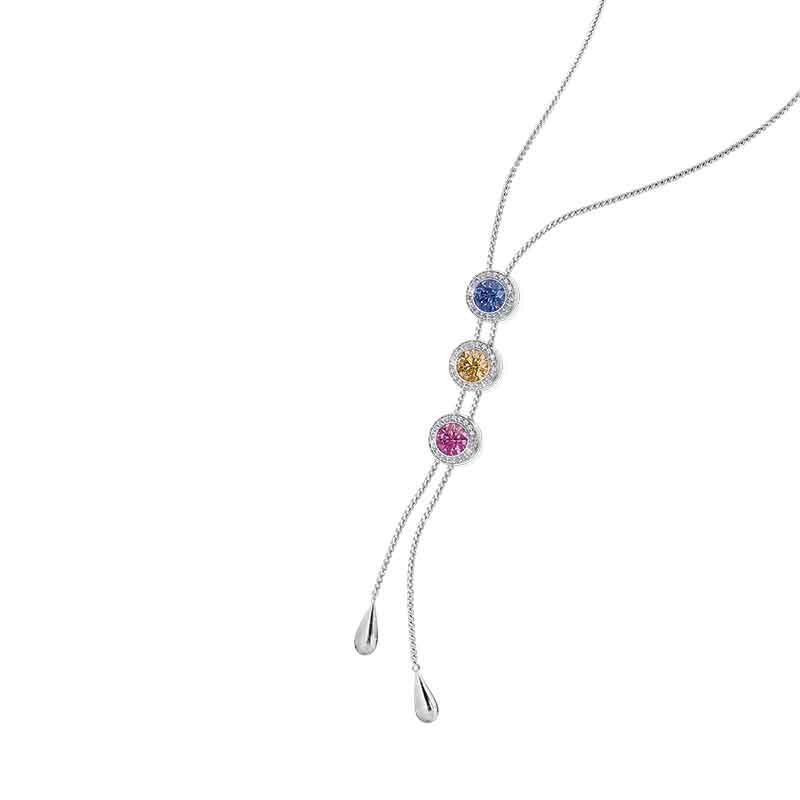Set against a white background, the image features an elegant, long necklace crafted from a fine silver chain. The chain is divided into two segments that originate from the upper right-hand corner and appear to almost meet in the middle before continuing downwards. At the ends of these strands are teardrop-shaped clasps, also in silver. The focal point of the necklace is its central section, where three round pendants are evenly spaced about an inch apart. Each pendant is encircled with small, sparkling diamonds. The top pendant features a blue gemstone, likely a sapphire or a blue crystal. The middle pendant showcases a golden yellow stone, possibly an amber or citrine, while the lowest pendant contains a pinkish stone. This intricate design gives the necklace a serpentine appearance, creating a stunning piece of jewelry.